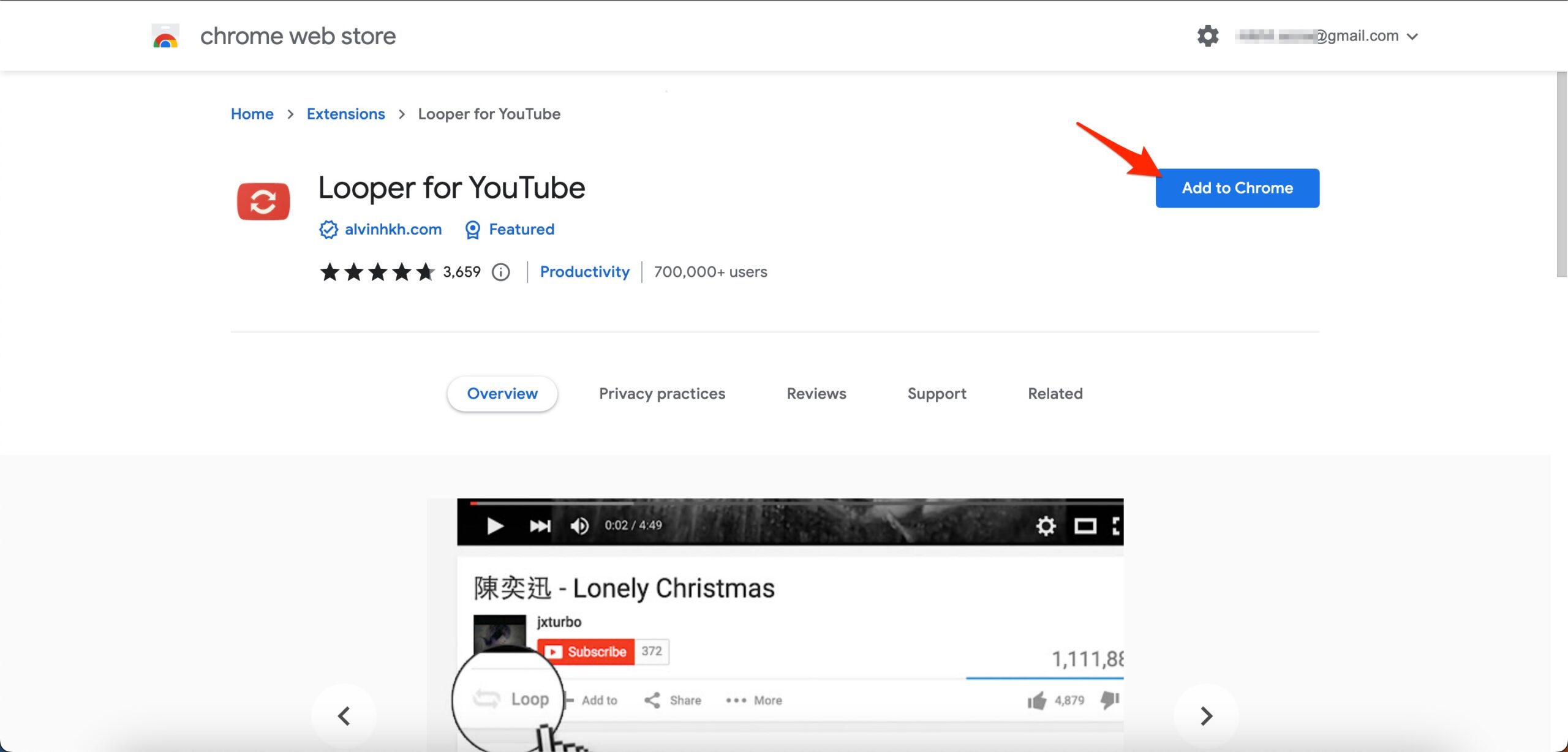This image is a detailed screenshot from the "Chrome Web Store" website. At the top left, there is a navigation bar displaying options like Home and Extensions. The focus is on an extension named "Looper for YouTube," as indicated by its red square icon with two curved arrows. Although the first part of the associated email address is blurred out, it is visible that the domain is at gmail.com.

The extension, named "Looper for YouTube" by AlvinHKH.com, is prominently displayed with a verification checkmark and a "Featured" badge next to it. Impressively, it boasts an average five-star rating from 3,659 reviews and falls under the "Productivity" category with over 700,000 users. A striking blue button labeled "Add to Chrome" is near the top and is highlighted by a red arrow pointing towards it.

Following this section, various tabs such as Overview, Privacy Practices, Reviews, Support, and Related are visible. At the very bottom of the screenshot is a partial thumbnail of a video titled "Lonely Christmas" in both Asian writing and English, uploaded by a user named JXTurbo who has 372 subscribers. The video has an icon indicating it can be looped, circled in black, with a pointer hovering nearby. Additional options like Plus Sign, Add to, Share, and More are also partially visible. The video has accrued 4,879 upvotes.